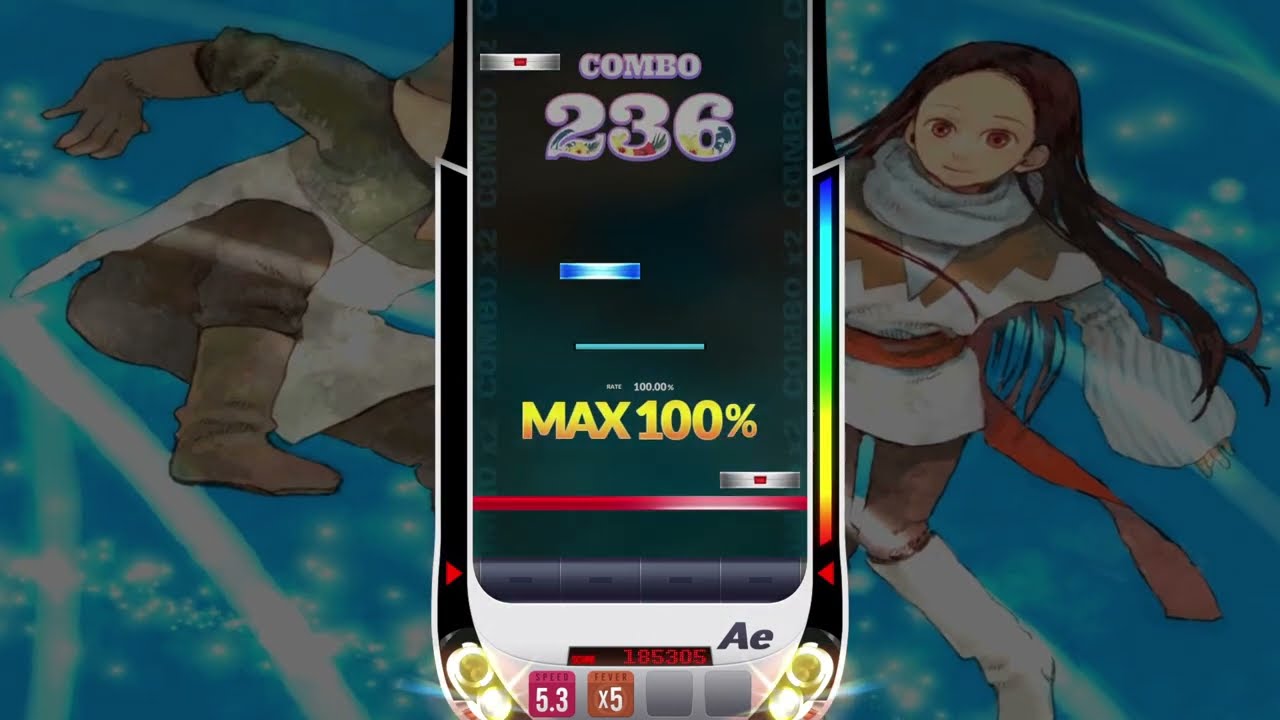In this detailed cartoon illustration, a white smartphone with a black screen sits prominently in the center, displaying "Combo 236" at the top in white text and "MAX 100%" in yellow at the bottom. The bottom of the screen also features "Speed 5.3 x 5" and the letters "AE" in the bottom right corner. The phone appears embedded in a clear or multi-colored cartridge that exhibits rainbow hues on the right-hand side and has some numbers near the bottom.

Behind the phone, the scene depicts an anime-style background resembling a blue sky with white lines and stars. On the left, a character clad in winter attire—including a brown and white sweater, brown pants, brown gloves, and brown boots—appears to be jumping or floating. On the right, a female anime character with large brown eyes and long dark hair is featured. She wears a white cowl-neck sweater styled like a tunic, black leggings, white knee-high boots, and a red sash. Both characters contribute to the fantasy-like, dynamic atmosphere of the scene, reminiscent of energetic video game graphics.